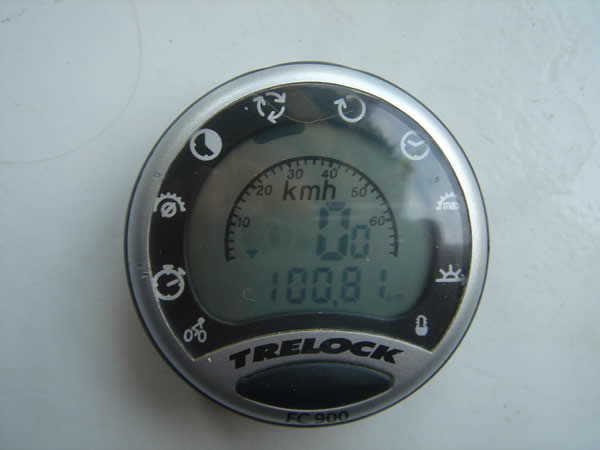The color photograph showcases a modern gauge set against a slate grayish-blue background. The circular gauge, bordered with a sleek silver outline, features a black inner ring adorned with an array of small white symbols, including arrows, an alarm clock schematic, a tiny bicycle, and a padlock. Beneath this, forming a crescent-like shape, is a metallic silver segment inscribed with the word "Trelock" (T-R-E-L-O-C-K). Occupying the central portion of the gauge is the actual dial, which intriguingly combines both analog and digital elements. The analog section is a semicircle marked with intervals of 10, ranging from 10 to 60, labeled as "K-M-H." The digital display prominently shows a large zero followed by a smaller zero, with a reading of "100.8" displayed below. The intricate details and clear markings suggest it measures speed and possibly other parameters.